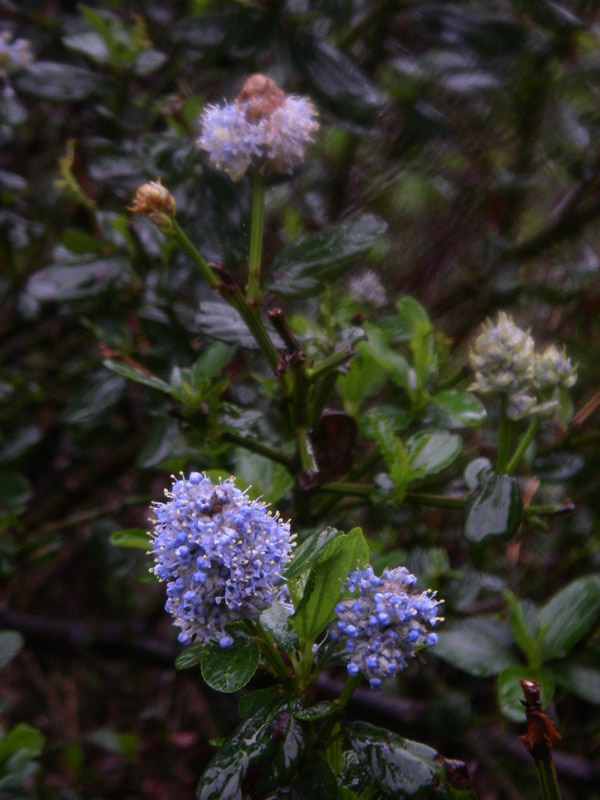This portrait-oriented photograph captures a detailed close-up of a bush featuring several tiny, purple flowers adorned with yellow hairs. The primary focus of the image is on two clusters of these flowers situated just below the center point. Each cluster is composed of small purple petals, which appear vividly clear against the darker, wet-looking green leaves surrounding them, suggesting a recent rainfall. The center of the top part of the image has another flower cluster, this one slightly faded and tinged with brown, indicating it might be wilting. Sun rays illuminate the scene, giving the wet leaves and flowers a glistening effect. The background is artistically blurred but reveals more leaves, flower buds, and potentially some small, unbloomed red and white flowers, all part of the same bush. This gives the image a shallow depth of field, emphasizing the intricate details of the highlighted flowers while suggesting the lushness of the garden surroundings.